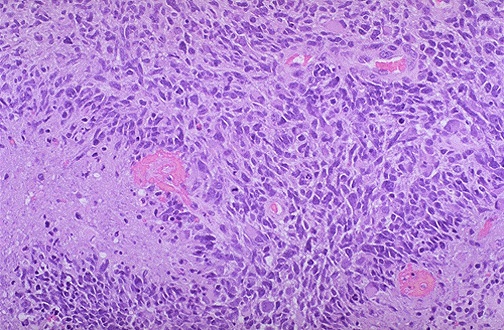The image presents a detailed, abstract close-up, reminiscent of a microscopic view of cellular structures. Predominantly light purple in color, it features twisting and curving shapes scattered throughout. These shapes vary, with many appearing circular or squarish in a deeper purple hue. Among this intricate pattern, there are distinct areas of light pink and larger circular pink blobs, notably positioned in the lower right-hand corner and the upper middle left-hand side. Additional light pink streaks intersperse the scene, and some regions near the top exhibit a lighter gray or white color, adding to the complexity. The overall composition gives the impression of magnified cells, with a honeycomb-like texture in some areas, though the exact nature of the structures remains ambiguous.